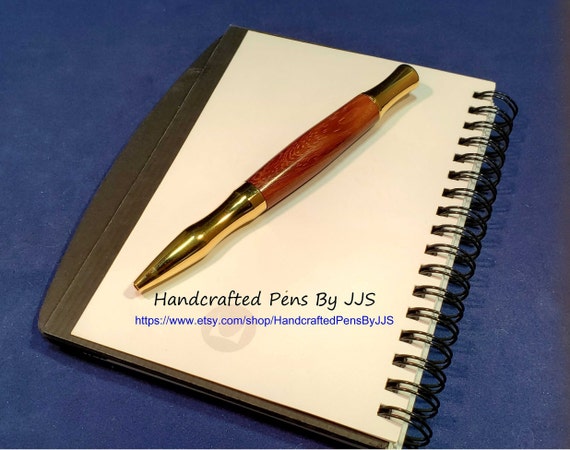The image depicts an elegantly staged advertisement for handcrafted pens by J.J.S. A luxurious, marbled reddish-rust colored pen with gold accents on both ends rests on an open spiral-bound journal. The pen features a narrow, cylindrical golden top and a similarly golden tip where one would write, with its distinct, fancy midsection being a standout feature. Inscribed beneath the pen is the text "handcrafted pens by J.J.S.," along with a website link to their Etsy shop, www.etsy.com/shop/handcraftedpensbyjjs. The journal, with either a black or brown cover, is open to a page that may be the first or last, where the advertisement is prominently displayed. This setup all rests on a navy blue background, possibly a table or countertop, adding to the sophisticated presentation of the product.